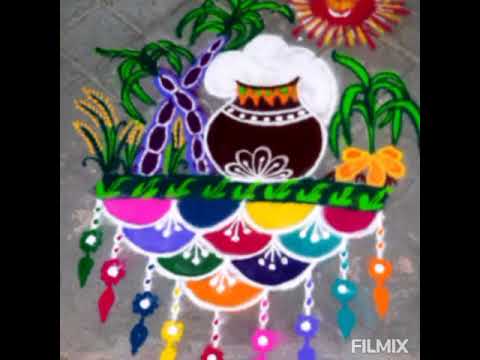This photograph captures a vibrant and intricately crafted Rangoli-style artwork against a gray terracotta tile background. The central piece is a black vase or cauldron with white smoke billowing out from its top, flanked by palm trees and positioned beneath a radiant red and yellow sun. This vase sits atop a grassy, leafy horizontal platform, adding a touch of nature to the artwork. The foundation of the display features a planter made of multicolored scalloped half-circles in hues of pink, navy, purple, red, green, orange, yellow, and turquoise, with a dark green rim adorned with bright green leaf patterns. Hanging from the bottom are colorful tassels or teardrop-shaped elements in shades of green, red, blue, yellow, pink, purple, turquoise, and orange, reminiscent of flowers or medallions. This lively arrangement is framed within a square format set against a black landscape-oriented background, with the text “FILMIX” in white at the bottom right, anchoring the piece in a contemporary context.